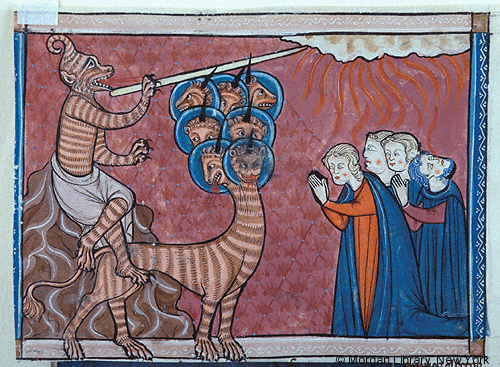This photograph captures an old-timey style painting with a unique border: blue with white squiggles on the left and right, and pink with white squiggles on the top and bottom, all encased in a white edge. The central scene portrays four kneeling, praying figures, one of whom looks up at the bizarre spectacle above them. Floating above them is a humanoid creature with gray, orange, and brown striped fur, adorned with a curly horn on its head, and wearing white shorts. It is depicted blowing onto a pointed stick which appears to interact with a cloud, causing a red stream to descend. Beneath this floating figure is a fantastical beast, covered in tan and white stripes, walking on four legs. This creature resembles a dragon or a possible tiger, featuring seven animalistic heads with blood streaming from their mouths, each head enclosed in glass domes and crowned with a single black horn, gazing in various directions. The bottom right corner bears the text “Copyright Morgan Library, New York,” adding an official timestamp to this intricate and evocative depiction.